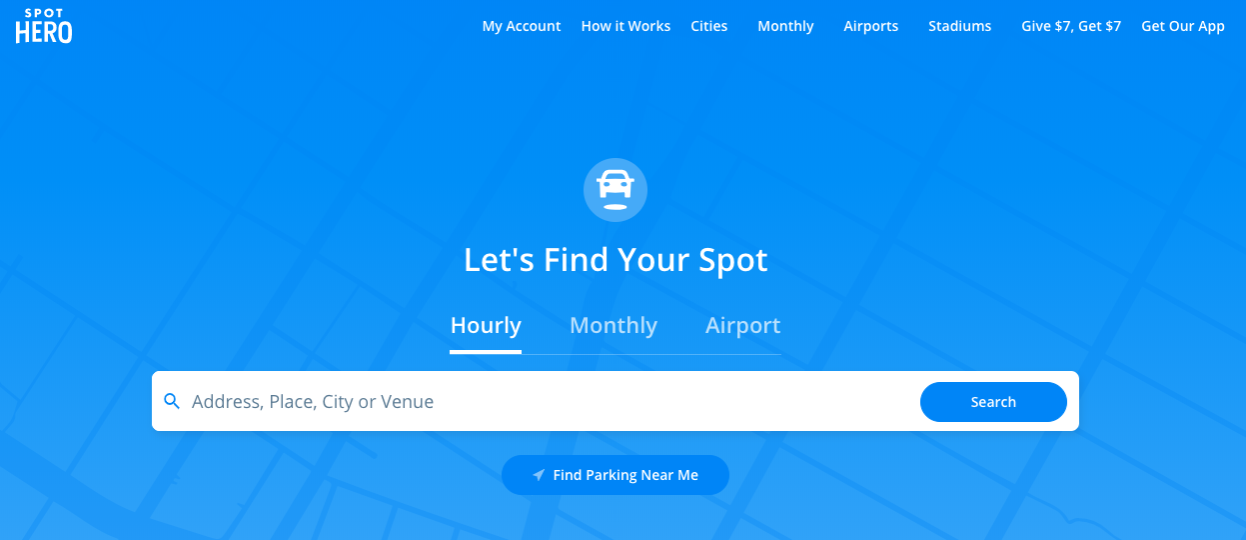The image depicts the top section of the Spot Hero website, framed against a blue background adorned with a faint, watermarked grid that resembles a city map. In the top left corner, the Spot Hero logo is prominently displayed. Across the upper portion, starting slightly left of the center, a white navigation bar lists various categories: "My Account," "How It Works," "Cities," "Monthly," "Airport," "Stadiums," "Give $7, Get $7," and "Get Our App." Central to the image is a graphic of a car, seemingly hovering above the ground, with a small circle beneath it that might represent its shadow or the ground. The main slogan, "Let's Find Your Spot," is also visible, followed by options like "Hourly," "Monthly," "Airport," "City or Venue," and a search function urging users to find parking spots. The overall theme suggests that Spot Hero is a service for renting parking spaces.